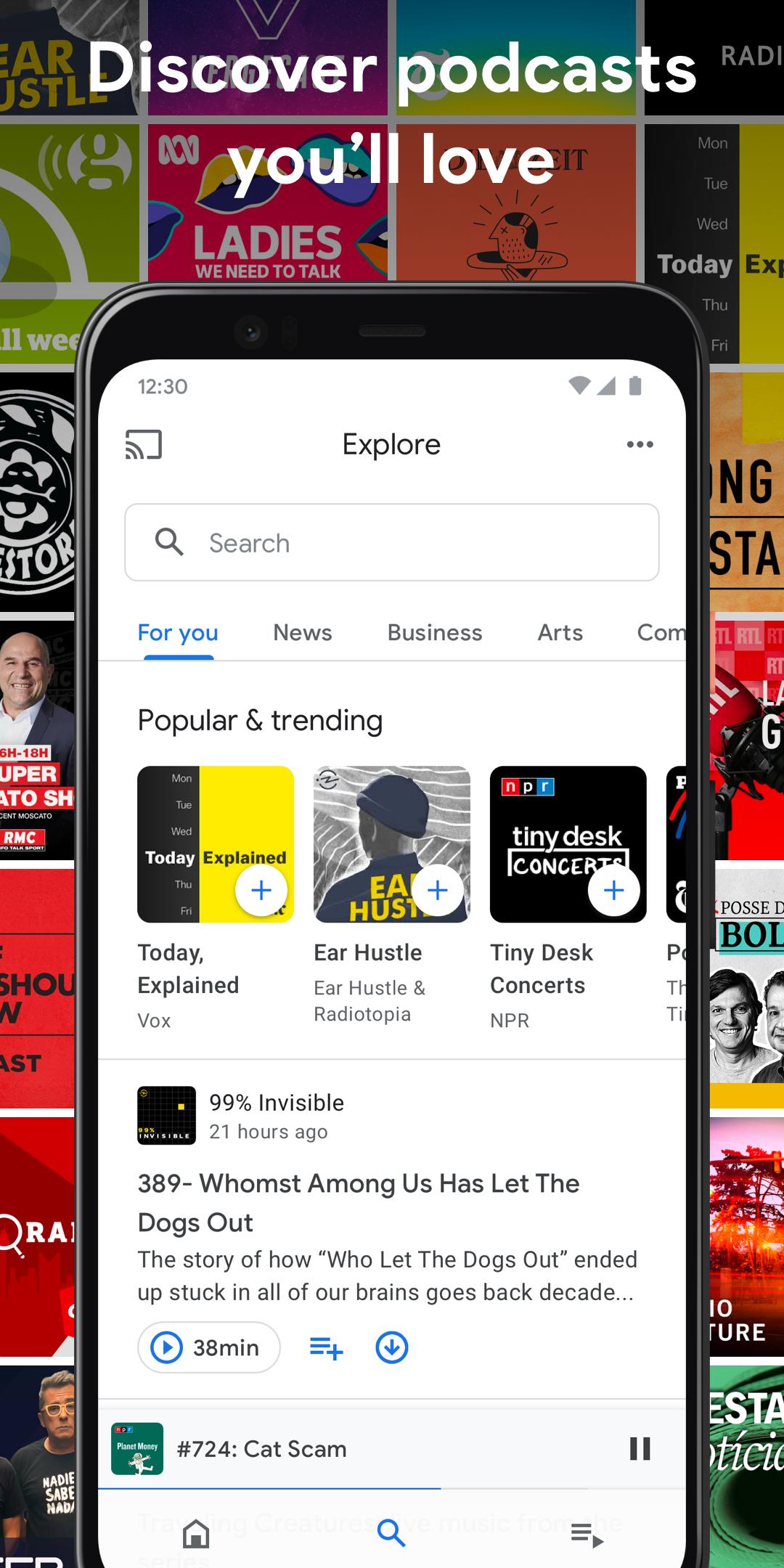The screenshot features a mobile interface promoting podcast discovery. At the top, a headline reads "Discover Podcasts You'll Love." Below, there is an image of a smartphone displaying the app's main interface. The screen shows a timestamp of 12:30 and an "Explore" option, along with a search bar containing a magnifying glass icon labeled "Search."

Underneath the search bar, there are several categories listed, including "For You," "London Blue," "News," "Business," "Arts," "Popular and Trending." Specific podcast episodes are highlighted, such as "Today Explained," "Ear Hustle," and "Tiny Desk Concerts," with the numbers "389" next to the title "Whomst Among Us Has Let the Dogs Out?" 

One featured episode explores the backstory of the song "Who Let the Dogs Out" and how it became ingrained in popular culture, clearly indicated by the text ending with an ellipsis "...". Additionally, there is a white oval with a blue play button and the number "38 min" displayed, indicating the duration of the episode. 

Other interface elements include three horizontal blue lines with a plus sign and a blue circle featuring a down arrow, as well as an episode labeled "#724 Cat Scam" accompanied by a pause button.